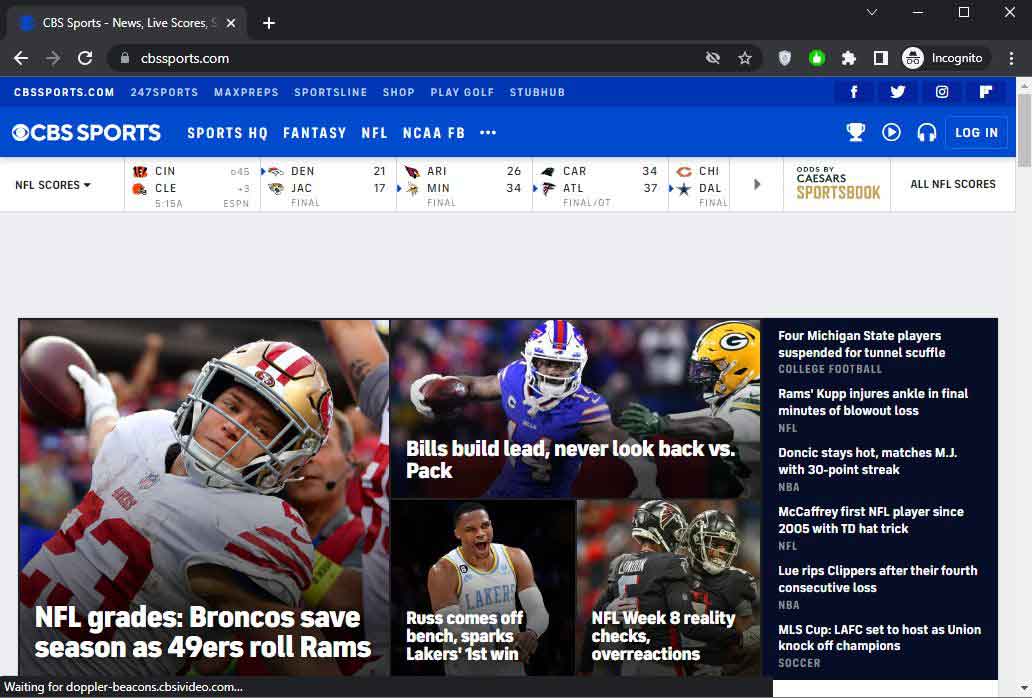The image displays a sports homepage on the website cbssports.com, viewed in incognito mode. The webpage header features a blue background with white text that includes the site name "cbssports.com." To the right of the site name are a series of clickable links including 247Sports, MaxPreps, SportsLine, Shop, PlayGolf, and StubHub. Additionally, there are social media icons for Facebook, Twitter, Instagram, and Fondo located on the far right.

Below the header, the CBS Sports logo is prominently displayed, followed by navigation links for Sports, HQ, Fantasy, NFL, NCAA, and more, extending into a series signified by ellipsis. Adjacent to these links are icons for a trophy, a play button, a headset, and a login button.

In the main content area, live scores for various sports games are displayed in a horizontal format. The scores include:
- Cincinnati 45, Cleveland 3 (at 5:15 a.m. ESPN)
- Denver 21, Jacksonville 17 (Final)
- Arizona 26, Minnesota 34 (Final)
- Carolina 34, Atlanta 37 (Final/OT)
- Chicago and Dallas are also listed, but their scores are not visible. Next to these is an indicator for "Odds by Caesars Sportsbook."

A clickable section labeled "All NFL Scores" is available. Below this, images and headlines for ongoing games and articles are shown:
1. "NFL Greats: Broncos Save Season as 49ers Roll Rams."
2. "Bill Lead Never Look Back vs. Pack."
3. "Russ Comes Off Bench, Sparks Lakers First Win."
4. "NFL Weekly Eight Reality Checks & Overreactions."

To the right, in a dark navy blue box, there are additional clickable links with corresponding headlines:
- "Four Michigan State Players Suspended for Tunnel Scuffle (College Football)."
- "Rams: Kupp Injures Ankle in Final Minutes of Blowout Loss (NFL)."
- "Doncic Stays Hot, Matches MJ with 30-Point Streak (NBA)."
- "McCaffrey: First NFL Player Since 2005 with TD Hat Trick (NFL)."
- "Lue Rips Clippers After Their Fourth Consecutive Loss (NBA)."
- "MLS Cup: LAFC Set to Host as Union Knock Off Champions (Soccer)."